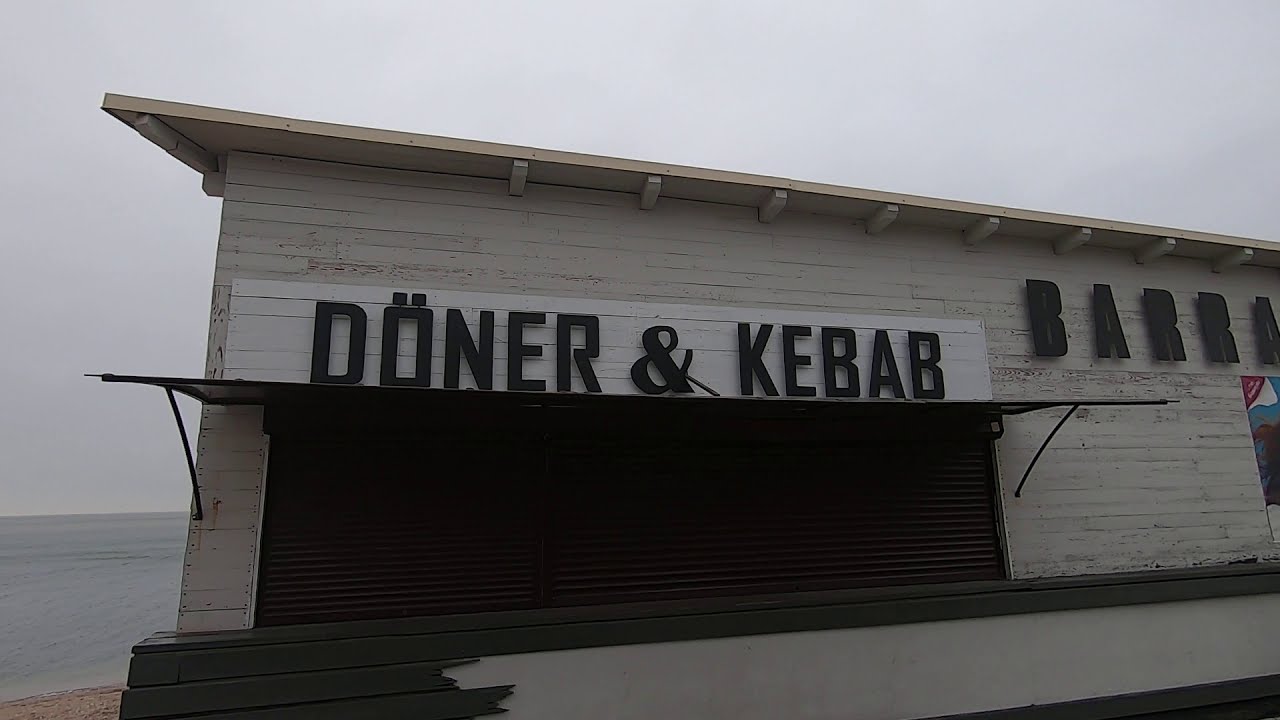The photograph captures an outdoor scene on a cloudy day with ominously dark clouds hinting at an impending rainstorm. Central to the image is a weathered, white-painted shack that appears to be a closed beachside snack shack. The structure, made of aged wood, features a black metal grate at counter height, rolled down to signal that the establishment is currently not in service. Above the counter is a small overhang, and above that, prominently painted in black letters on the white façade, is the name of the business: "Donor & Kebab." 

Further details reveal another set of partially visible black letters to the right, forming "B-A-R-R-A," hinting at an additional word or name not fully captured in the photo. The shack's chipped paint and some broken boards expose the white stucco material beneath, adding to its rustic appearance. Positioned on the corner of the building, the viewer can glimpse behind it to a rocky beach and a body of water to the left, contrasting the scene with a touch of natural beauty. The overall clarity of the image ensures that even these fine details are perceptible, all under a naturally lit, daytime setting.